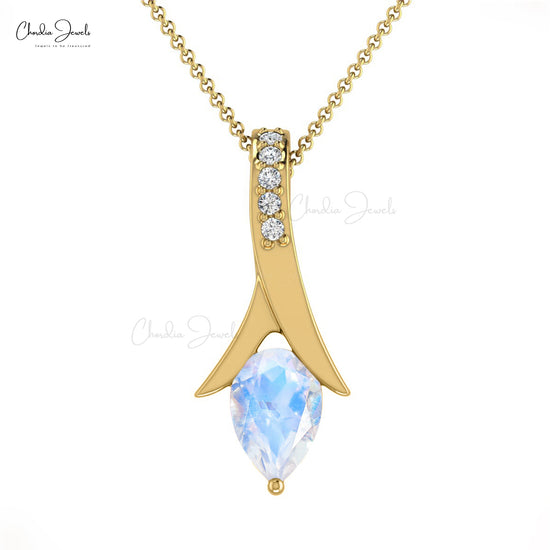This photograph showcases a luxurious gold necklace, prominently featuring a V-shaped chain segment. The centerpiece of the necklace is an intricately designed pendant, also crafted from gold, which forms an elegant upside-down Y. Adorning the upper part of the Y are five sparkling diamonds, which add a touch of brilliance. Dangling from the bottom of this pendant is a teardrop-shaped diamond with striking blue accents, further enhancing its allure. The pendant also incorporates a tiny gold circle at the very bottom, adding a subtle yet exquisite detail. Additionally, the image contains an inscription of someone's name in cursive, although it is too small to decipher.